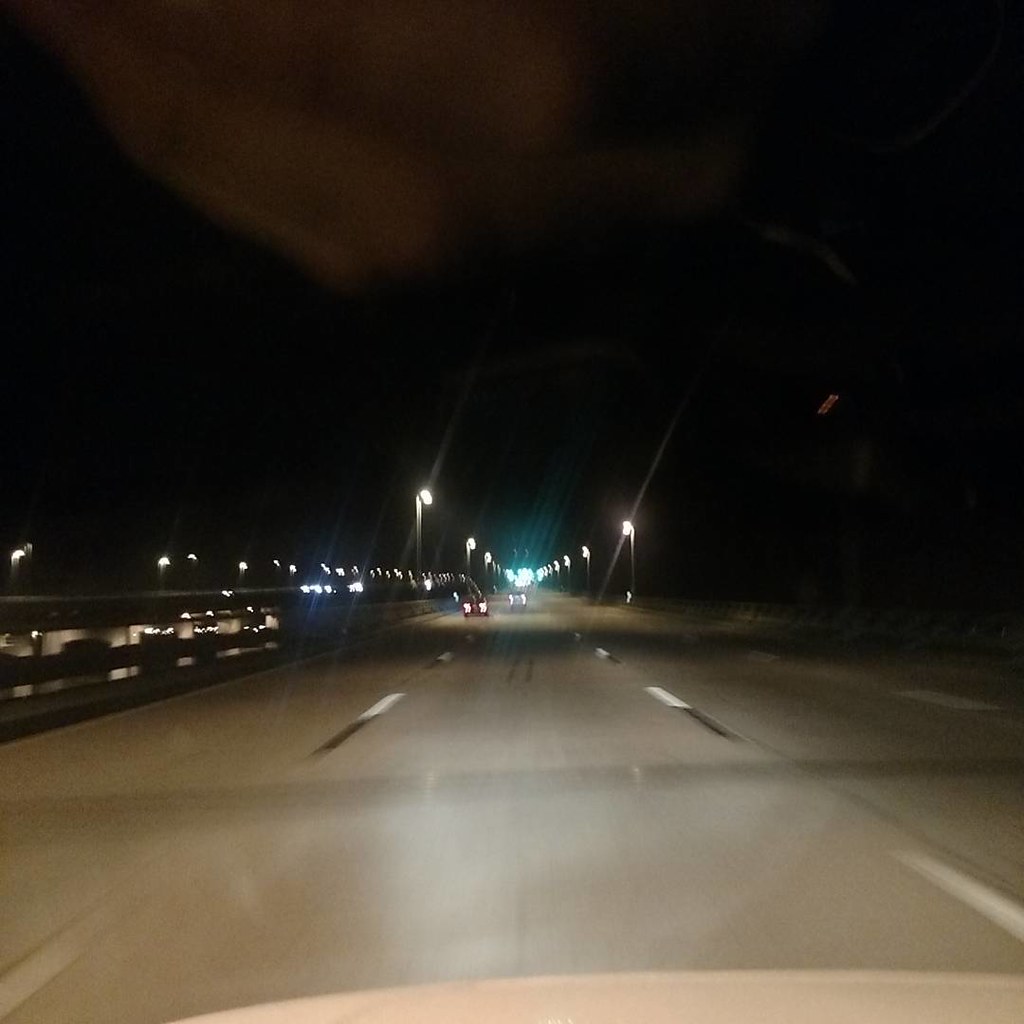A slightly blurred nighttime photograph taken through the windshield of a moving vehicle captures a major three-lane highway, illuminated by evenly spaced streetlights and the vehicle's headlights. The road is demarcated with white markings along its outer edges, guiding the way through a pitch-black sky devoid of buildings. A bridge structure emerges on the center left, adding an architectural element to the scene. The lower part of the image subtly reveals the hood of the vehicle, suggesting it is white or light-colored. The composition conveys a sense of solitude and motion, typical of late-night drives on expansive highways.